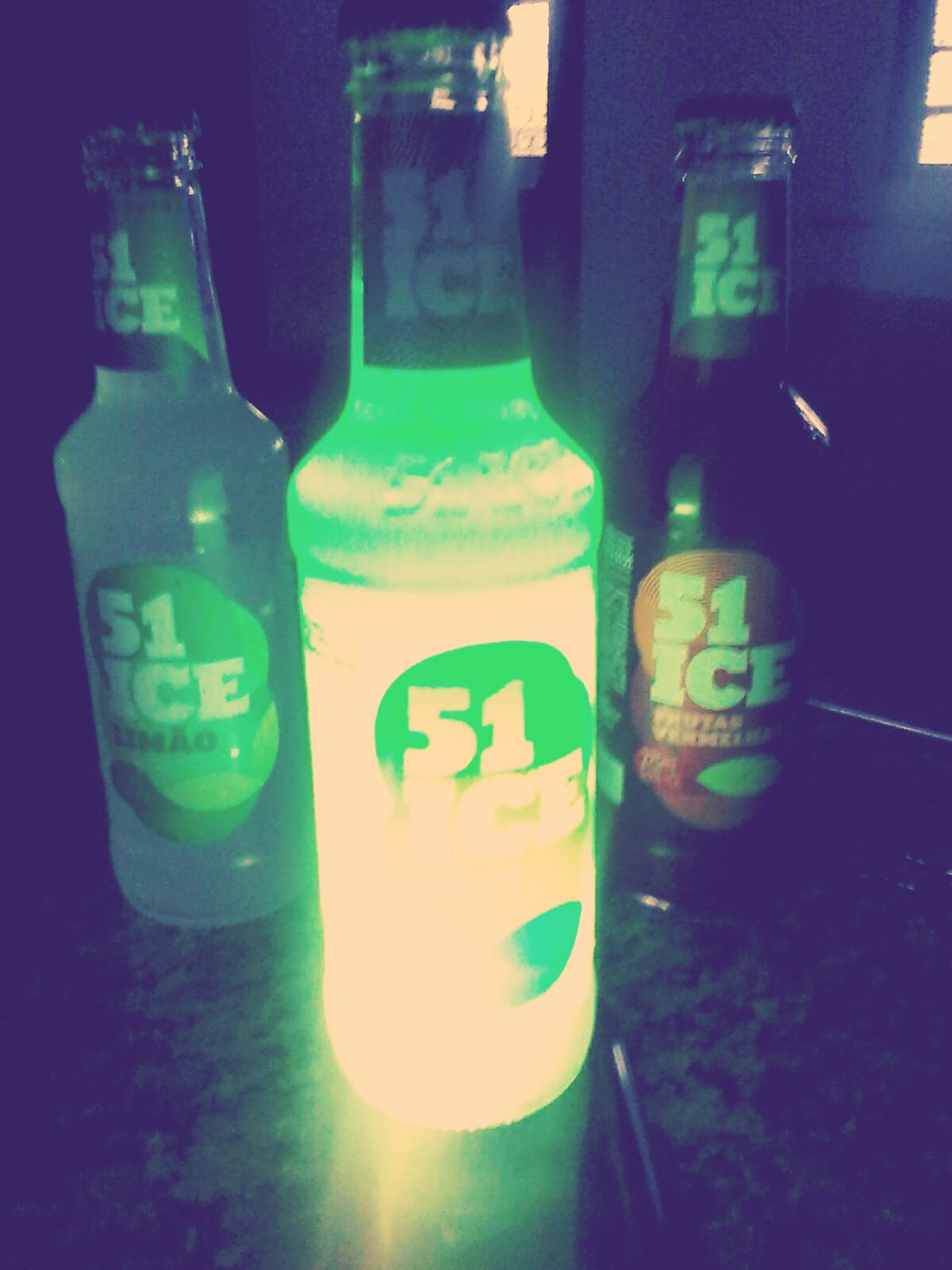The photograph captures a trio of unopened beverages placed centrally on a dark, glossy countertop, possibly in a nightclub. The setting is predominantly dark, with the only notable background details being two dimly lit windows. Each bottle features a prominent label bearing the text "51 ICE" in bold white capital letters, suggestive of a flavored soda or perhaps an alcoholic drink. The central bottle stands out dramatically, illuminated from a neon green backlight that imbues it with an almost glowing appearance, making the label difficult to read. This stark lighting casts a green reflection onto the countertop below. In contrast, the flanking bottles are in relative darkness but still distinguishably labeled. The left bottle has a green circular label, while the right bottle's label has a brown hue. The vibrant green, black, and white hues dominate the scene, enhancing the nightclub-like ambiance.